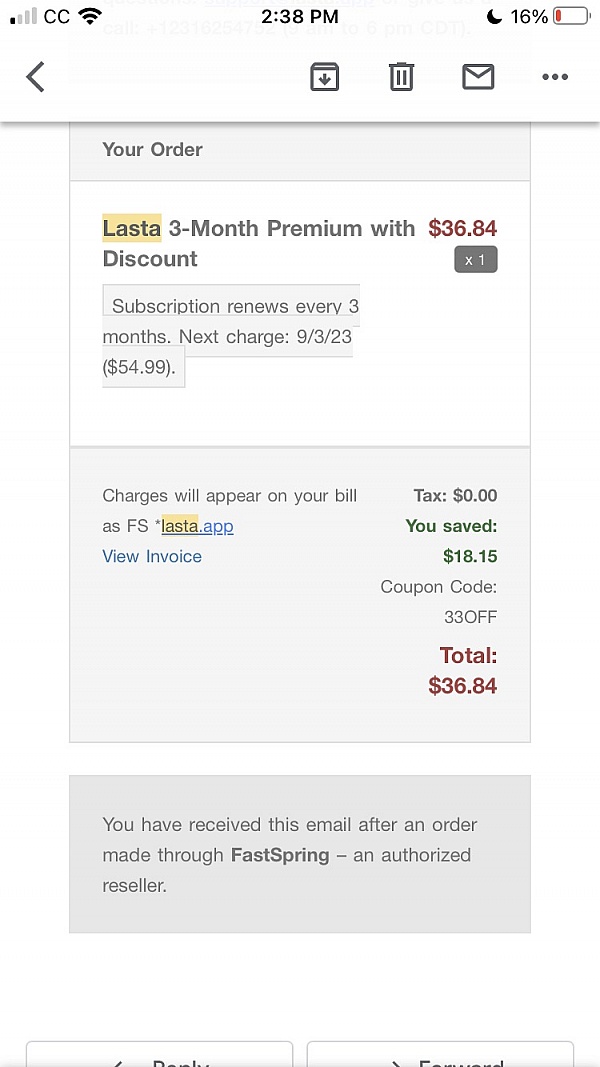This image appears to be a partial screenshot taken from an iPad or mobile phone, as indicated by several elements in its interface. In the top left corner, there is a signal bar displaying low signal strength, and the letters "CC" next to it. Adjacent to this, the time is shown as "2:38 PM". Moving right, there is a crescent moon icon, suggesting a "Do Not Disturb" mode, followed by a "16%" battery indicator with a low battery symbol featuring a red dot.

Below this status bar, there are several icons: a left-pointing arrow, a square with a down arrow, a trash can, an envelope, and a set of three horizontal dots. Under this row of icons, a gray bar is labeled with "Your Order."

The main content includes a white box highlighted in yellow which reads "LASTA," indicating a "three-month premium with discount" for $36.84 with a quantity of one. It details that the subscription renews every three months, with the next charge being $54.99 on 09/03/23. 

Beneath this, another gray box gives further details, stating, "Your Charges will appear on your bill as F-S * LASTA.app, view invoice", followed by tax information showing $0.00, a savings of $18.15 due to a coupon code "33OFF", and a total charge of $36.84.

Further down, a gray box notes, "You have received this email after an order made through FastSpring, an authorized reseller." At the bottom of the screenshot, two partially visible white buttons, labeled "Back" and "Forward," are cut off by the image's edge.